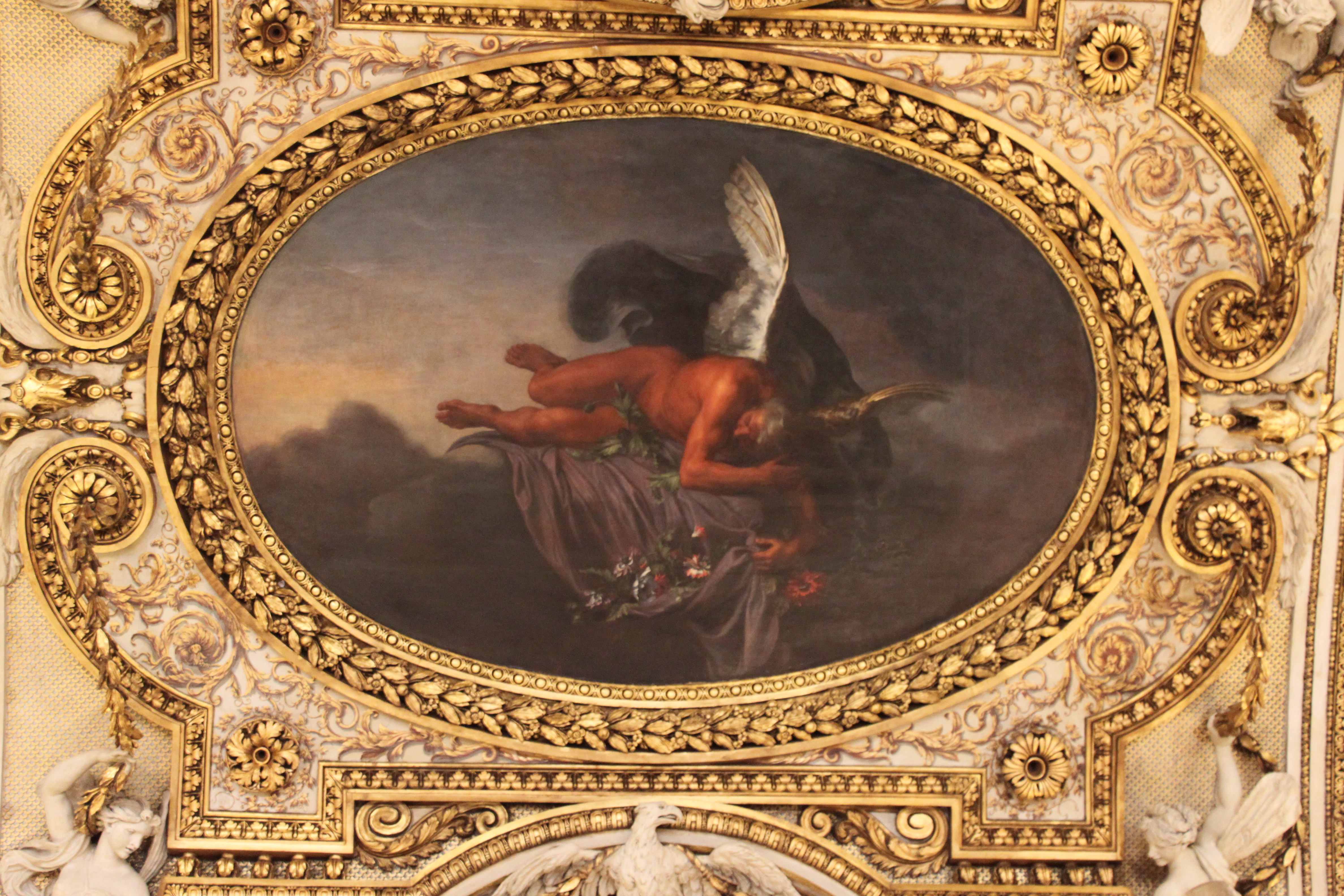The image captures a highly ornate and intricate scene that seems to be the ceiling of a grand church or cathedral. Dominating the center is a large oval painting bordered with elaborate gold filigree and leaf patterns forming a grand oval shape. Surrounding this central piece are numerous Gothic circular designs, thorns, and floral motifs, giving it a rich, decorative appearance. Flanking the oval on either side are white statues of angels, positioned at the bottom left and bottom right corners of the image. Directly beneath the oval rests an imposing statue of an eagle.

Inside the oval, the scene becomes even more dramatic and evocative. It depicts an enigmatic winged figure, possibly a demon or a dark-skinned angel with white wings, reclining on a platform draped with a purple cloth adorned with flowers. The figure lies amidst a cloudy backdrop, with gray clouds enveloping him, giving the impression that he is floating in the sky. A dark, mist-like form looms behind the figure, adding to the mystical and somewhat foreboding atmosphere. The detailed contrast between the ornate golden surroundings and the tranquil yet mysterious central scene creates a captivating visual narrative.